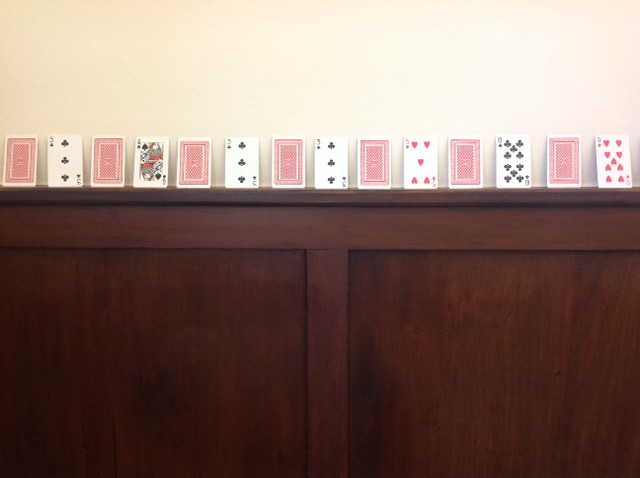In the image, the lower two-thirds prominently feature a dark cherry or walnut-stained headboard, divided into two symmetrical panels by a vertical one-by-four plank at the center. This central plank connects to another horizontal one-by-four board running along the top of the headboard, which is adorned with a decorative top shelf. 

Resting on this top shelf, against an off-white wall, are fourteen playing cards meticulously balanced in an alternating pattern of card backs and faces. Starting from the far left, the first card presents the classic red back of a standard playing card deck, followed by the three of clubs, another red back, the queen of clubs, and so forth. The visible card faces are the three of clubs (appearing three times), the queen of clubs, the five of hearts, the ten of clubs, and the nine of hearts, interspersed with red-backed cards.

The repetition of certain cards, such as the three of clubs appearing thrice, indicates that these cards are sourced from multiple decks or a specialized deck that includes multiple instances of the same card.